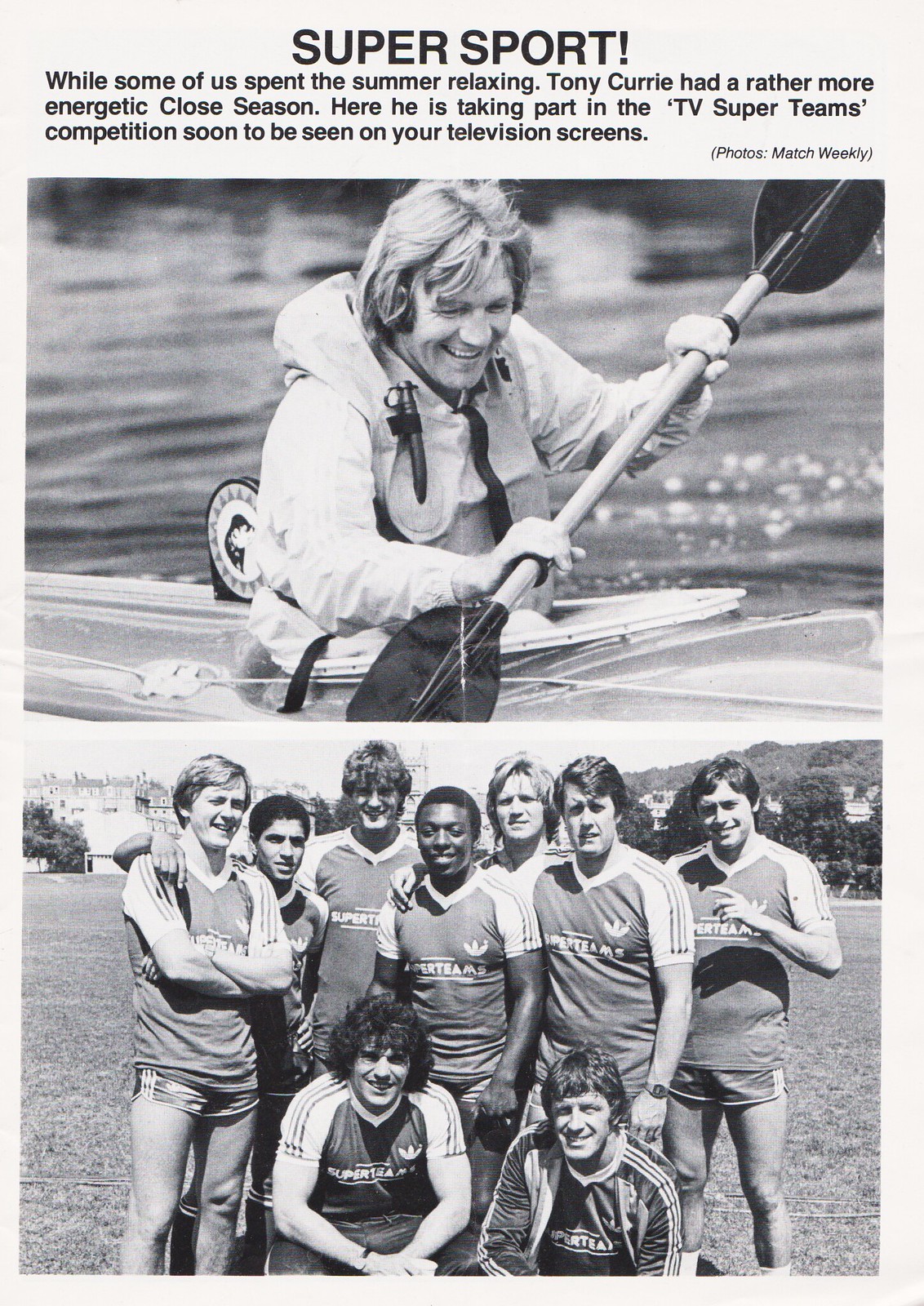In this detailed black-and-white magazine page, the title "Super Sport!" is vividly printed at the top in bold black ink on a white background. Below the title, the caption reads, "While some of us spent the summer relaxing, Tony Currie had a rather more energetic close season. Here he is taking part in the TV Super Teams competition, soon to be seen on your television screens."

The page features two black-and-white photographs. The top photograph is a close-up of a blonde-haired man, identified as Tony Currie, smiling as he holds a double-sided paddle. He is seated in a kayak, surrounded by water and wearing waterproof gear with a hood. The bottom photograph captures a group of nine men, all wearing athletic uniforms consisting of short-sleeved shirts labeled "Super Teams" and shorts. They are outdoors on a grassy field, with two men kneeling in the front row and seven standing behind, all smiling at the camera. The background includes grass, trees, a hill, and some sort of building. Both photographs are credited to Match Weekly.